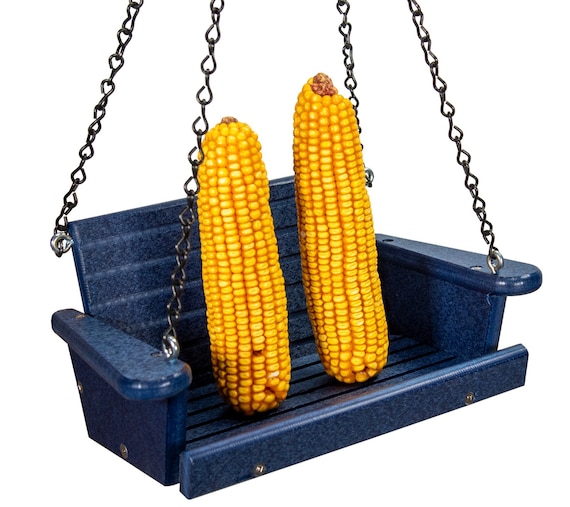This color photograph showcases a miniature garden swing, painted in a navy blue hue, seemingly designed as an ornament rather than a functional seat due to its small size. The swing is meticulously crafted from wood with slatted details and is suspended by four rusty silver metal chains extending beyond the image frame. The scene features two dried corn cobs positioned side by side on the swing, leaning against its backrest, portraying a whimsical touch as if they were a couple enjoying a peaceful moment together. The entire setup is placed against a stark white background, emphasizing the playful and decorative nature of the piece. Notably, there are two visible screws on both the front and the sides, adding to its quaint, handcrafted appeal.